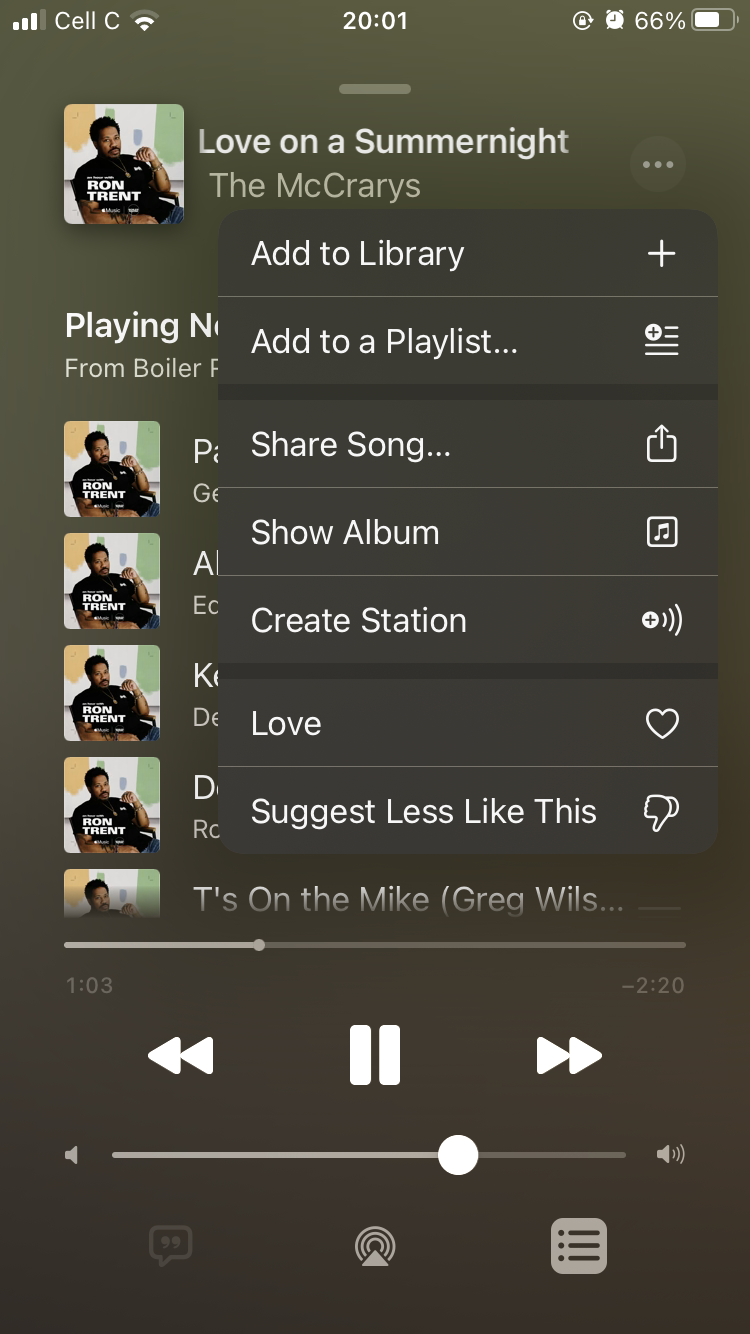A detailed screenshot from a music app on a mobile device. At the top of the screen, various phone icons are displayed, including four bars indicating cellular signal strength, the "cell C" network, a Wi-Fi symbol, the time reading 20:01, a clock symbol, and a battery icon showing 66% charge. The central part of the screen features an image of Ron Trent – a black man seated in a chair, wearing a black shirt and blue pants, adorned with jewelry, including a necklace and bracelets. He sports a black mustache and is looking directly at the camera. His name, "Ron Trent," is written in white text above the image. Below his picture is a playlist of his songs, with the first song being "Love on a Summer Night" by The McCrarys. A pop-up menu partially covers the song list, offering options such as "Add to Library," "Add to a Playlist," "Share Song," "Show Album," "Create Station," "Love," and "Suggest Less Like This." At the bottom of the screen are standard music playback controls, including a rewind icon, pause button, and fast-forward icon, along with a progress bar and a circular indicator showing the current position of the song being played.